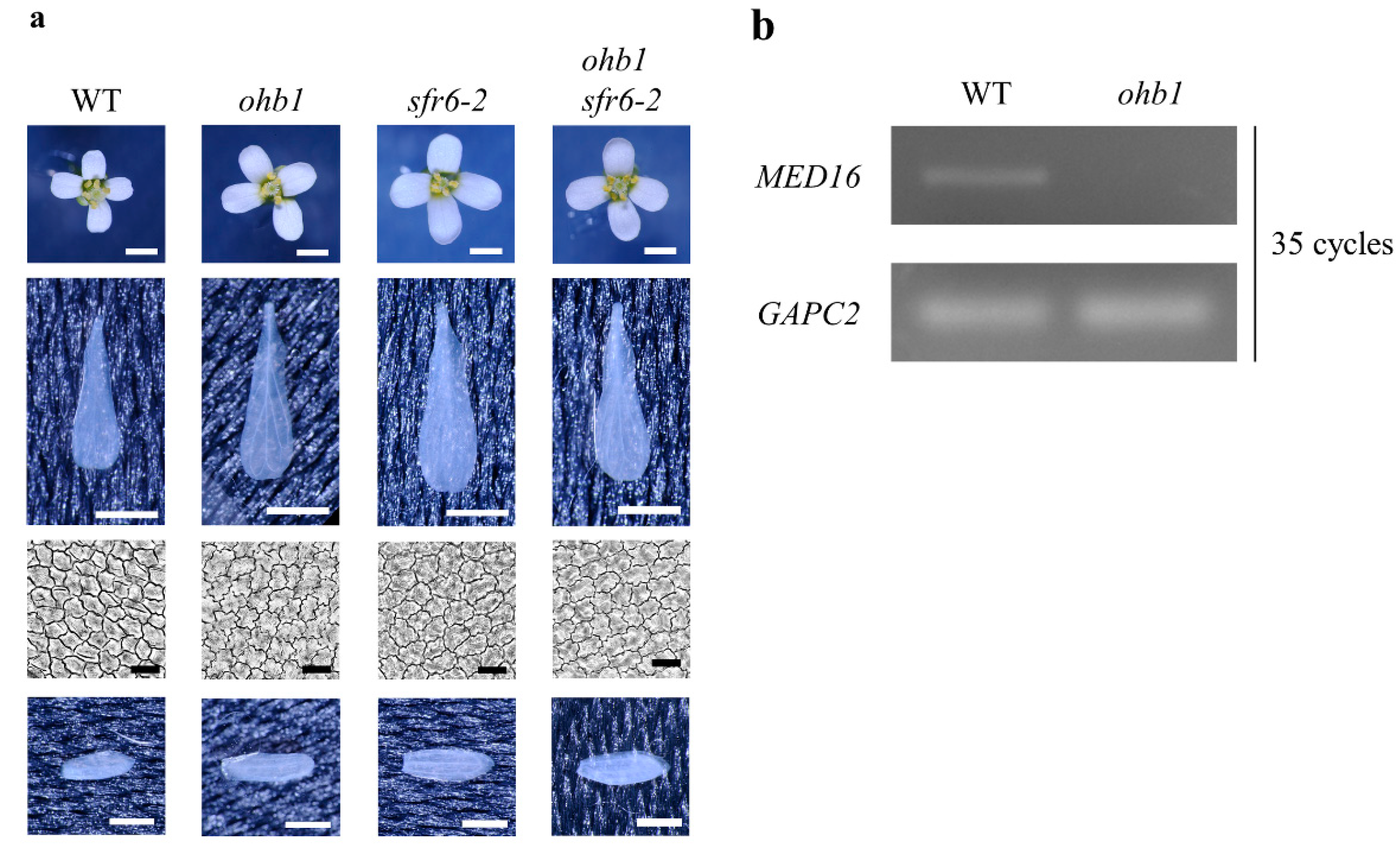This image is a composite of 18 individual images arranged in a grid with four columns on the left and two bars on the right, all separated by white borders. The image is predominantly square with no external border, set against the white backdrop of the screen. At the top of the columns on the left, small letters 'A' and 'B' label the upper left and right respectively. Each column and row is further labeled with specific text: the first column labeled 'WT', the second and fourth columns labeled 'OHB1', and the third column labeled 'SFR6-2'.

The first row features four progressively larger white flowers with yellow centers on blue backgrounds. The second row contains teardrop shapes in light blue against darker blue backgrounds. The third row displays gray scale images that resemble cells. The fourth row mirrors the blue background of the second row but with pill-shaped light blue ovals. To the right, there are two horizontal gray bars labeled 'MED16GAPC2' on the left and '35 cycles' on the right.